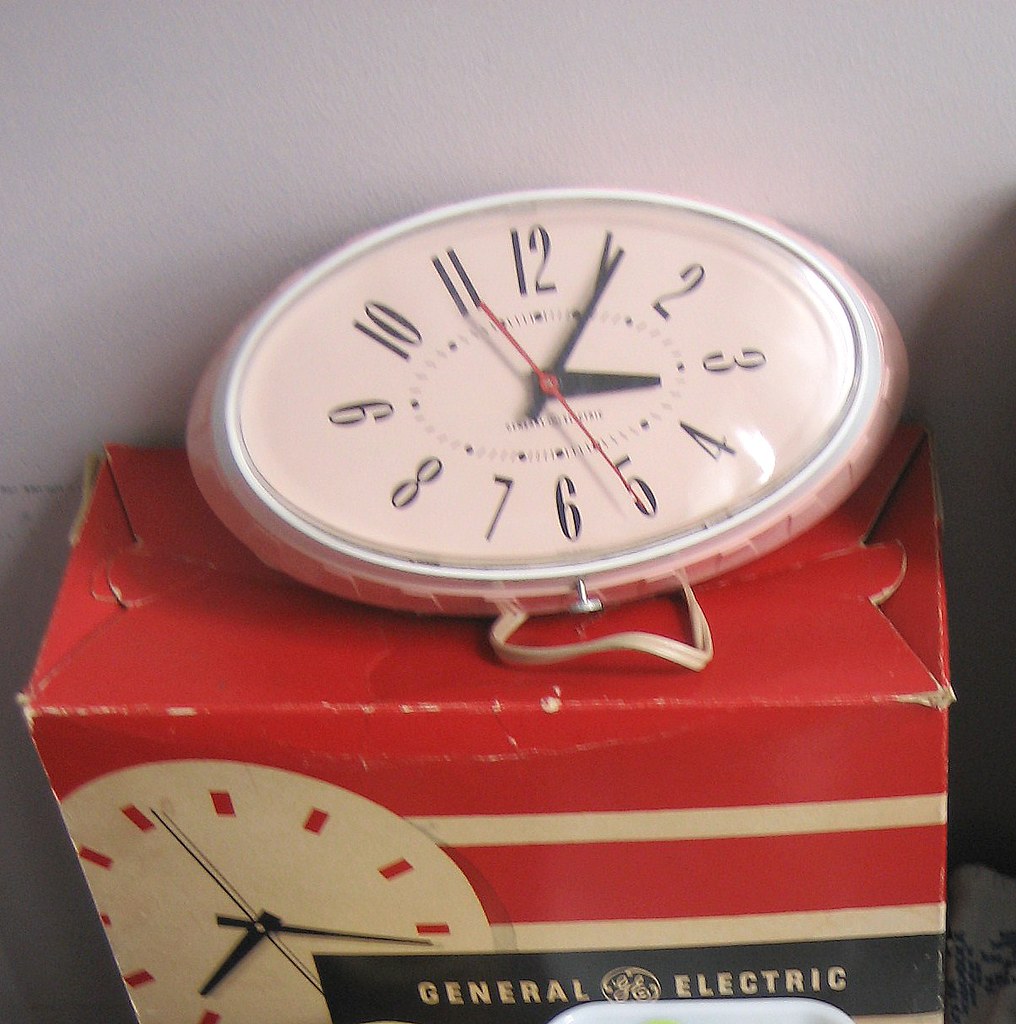A detailed image shows an oval clock face resting atop a box. The clock features a white background with contrasting black numerals and a black hour and minute hand, complemented by a red second hand. The time displayed is 3:06. Extending from the bottom, near the six o'clock position, is a white-tan band, suggesting the clock is part of a wristwatch configuration. This area also includes a small silver winding dial. The clock sits on a predominantly red box that bears the "General Electric" brand name in black and off-white text, set against a black background. The left side of the box has an image of the clock. There are noticeable shadows on the left side of the photograph, which along with the clock and box, is placed against a gray wall.